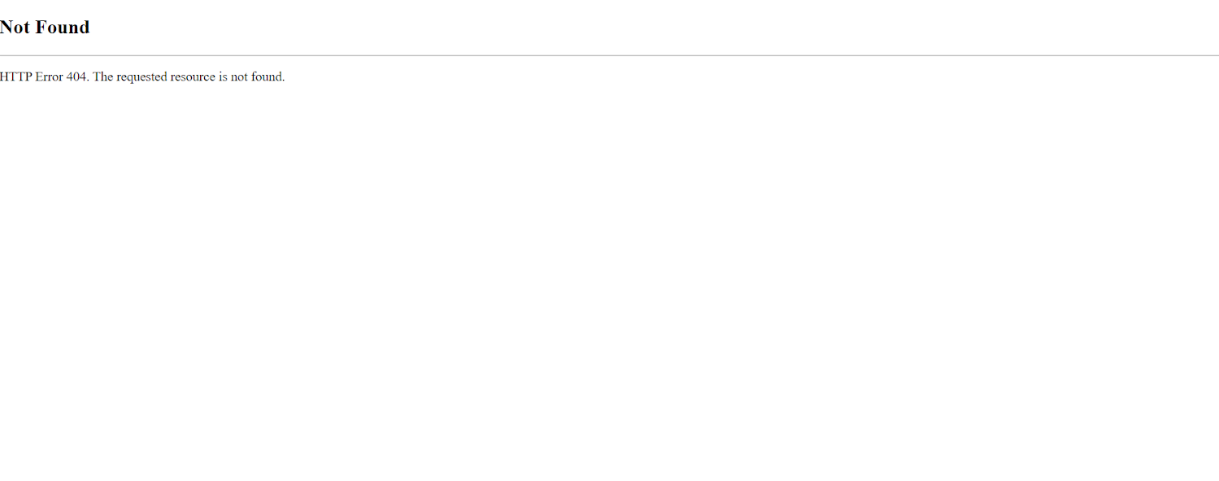The image depicts a desktop screenshot, characterized by its large width. Dominating the image is a predominantly white background. Prominently positioned at the top center in bold black title case text are the words "Not Found." Below this text runs a thin, uninterrupted black line stretching across the entirety of the width. Under the line, additional text in black reads: "HTTP Error 404. The requested resource is not found." This message indicates that the website failed to load properly due to a missing resource. The Hypertext Transfer Protocol (HTTP) error code 404 signifies that the resource could not be located, although it does not specify whether the absence is permanent or temporary. The user might resolve this by checking other parts of the website, reloading the page, or trying again at a later time.